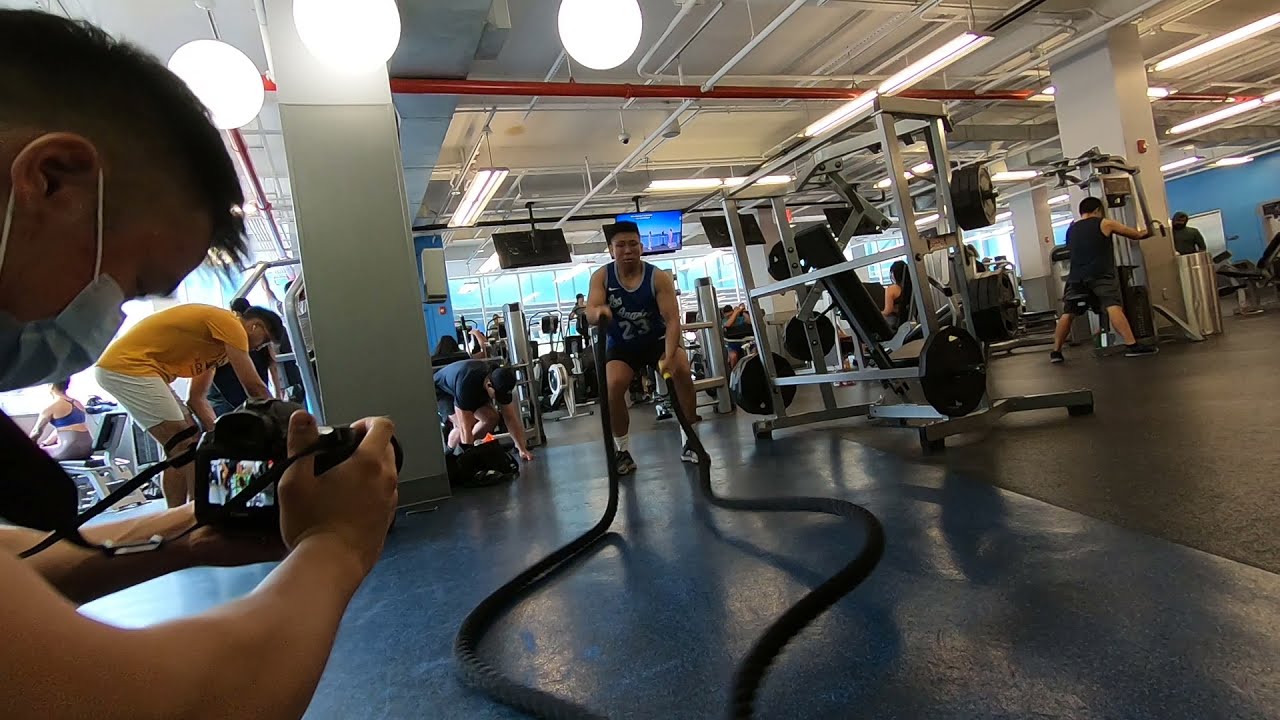This photograph captures the dynamic atmosphere of a gym. Central to the image is a man standing on a blue mat, wearing a distinctive blue and white Los Angeles Lakers LeBron James jersey, marked with the number 23 and the Nike swoosh. He pairs this with blue shorts and tennis shoes. Firmly gripping a thick black rope with yellow handles in each hand, he is engaged in an intense rope workout, rhythmically moving his arms up and down. Surrounding him, several other gym-goers can be seen utilizing various pieces of equipment, indicating a bustling yet orderly environment. To the left, a man with short black hair and a light blue face mask holds a black camera, possibly recording the workout session. The gym’s flooring features sections of blue mats and gray carpeting, while the white ceiling, supported by pillars and lit with large fluorescent lights, adds to the bright and energetic setting. Additionally, gym equipment and weights are scattered around, contributing to the active ambiance.